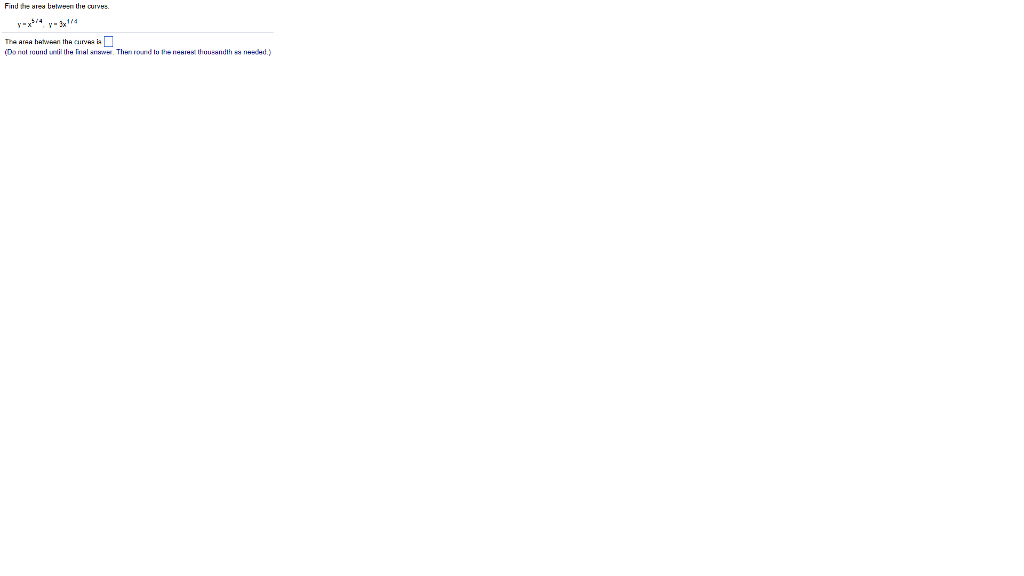Here is a detailed and cleaned-up caption for the described image:

---

This image is quite small, comparable to the size of a thumbnail, and required zooming in to decipher its content. At the top, in black text, there is a prompt that reads, "Find the area between the curves." Below this, the following mathematical formulas are provided:
- \( Y = X^{5/4} \)
- \( Y = 3X^{1/4} \)

A light-colored gray line runs horizontally from left to right beneath these formulas. Further down, in black text, there's an instruction that states, "The area between the curves is," followed by an empty white box outlined in blue, presumably for the answer to be inserted. Additionally, there is a note in blue, parenthetical text advising, "Do not round until the final answer; then round to the nearest thousandth as needed." The background of the image is entirely white, maintaining uniformity with the rest of the page.